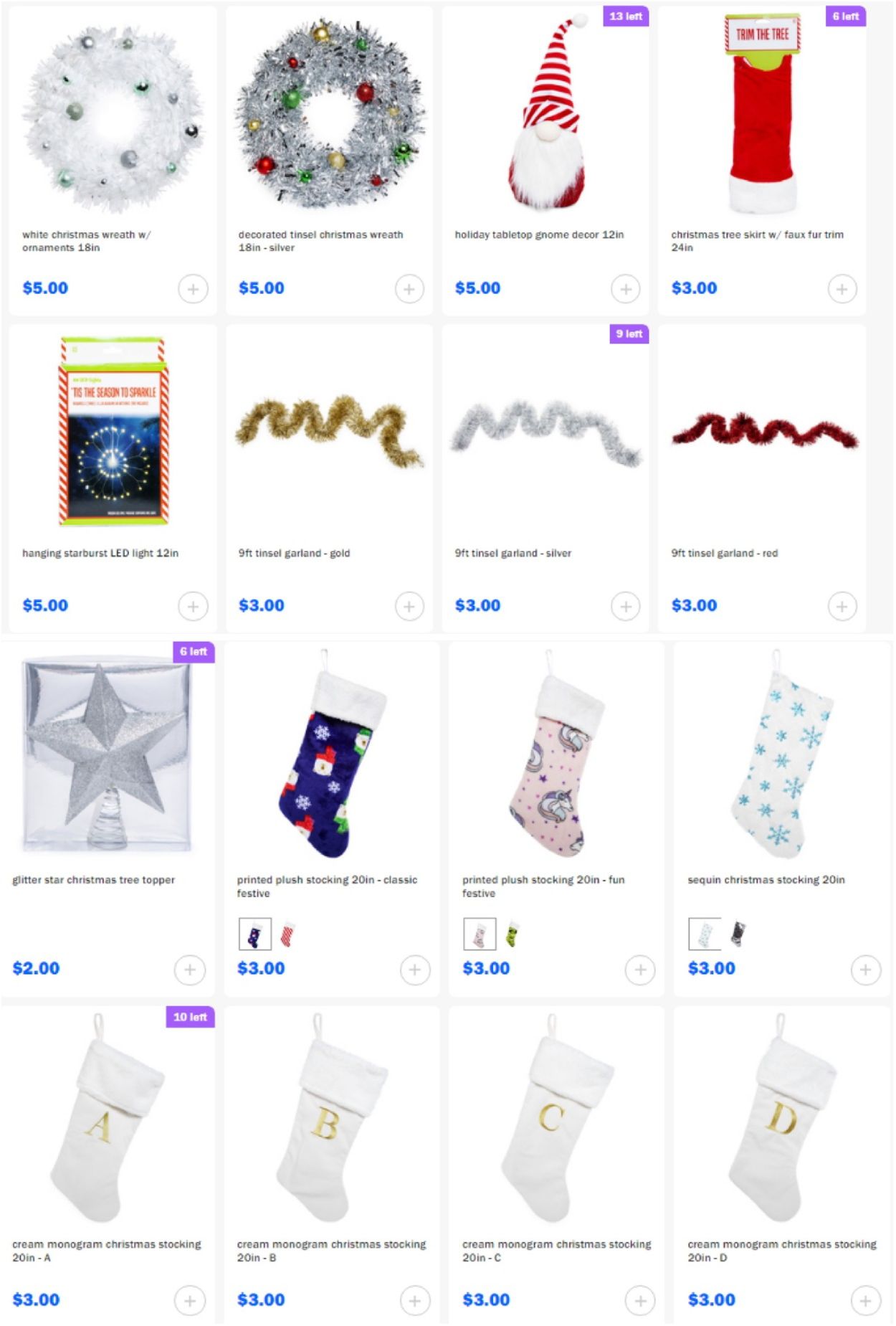This image showcases a Christmas-themed e-commerce website featuring a variety of festive items displayed in individual boxes against a white background. The top row includes two Christmas wreaths—one in white and the other in a silver color adorned with red, green, and gold baubles. Prices are visible but quite blurry, estimated to be around $5 each. Adjacent to the wreaths is an image of a gnome, also priced at approximately $5.

On the second row, there is a traditional Santa hat priced at $3. Next to the hat, there's a somewhat indistinguishable item intended for hanging, though the description remains unreadable. Following this, two varieties of garland are displayed, featuring colors of gold, silver, and red.

Further down, a star-shaped tree topper is prominently featured. The remaining items include an assortment of Christmas stockings in various colors and designs. These include a blue stocking, a pink stocking, and a white stocking with blue designs. At the bottom of the website, additional white stockings are labeled with gold lettering, each marked with the letters A, B, C, and D.

Overall, the image offers a cheerful preview of holiday decorations, perfect for sprucing up any Christmas setting.